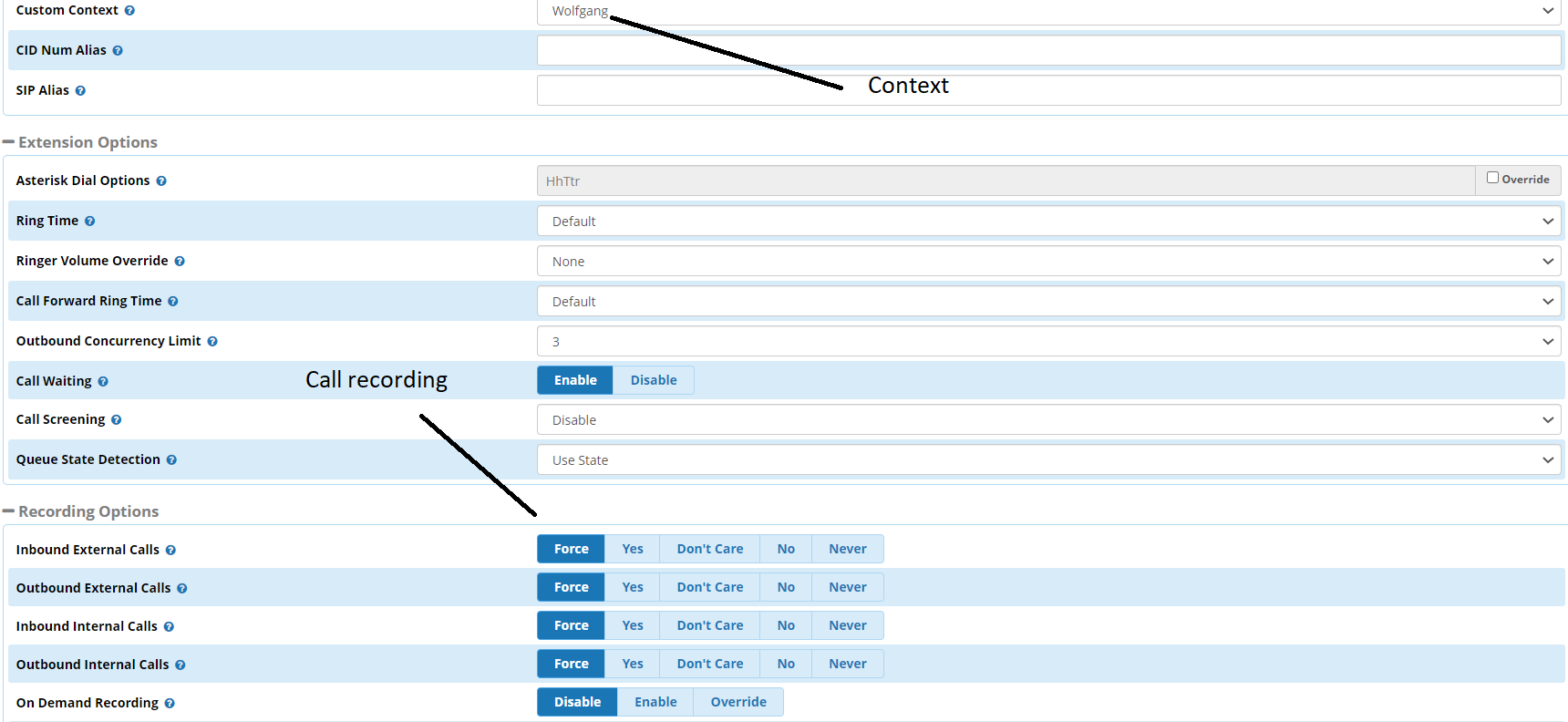The image features a detailed chart split into two sections: a main display and a smaller tab on the side.

### Left Section:
This section is primarily composed of various categories and their corresponding parameters, color-coded for differentiation:
- **Custom Context**: 
  - CID Number (Blue)
  - SIP Alias (White)
- **Extension Options**: 
  - Asterisk Dial Option (White)
  - Ring Time (Blue)
  - Ringer Volume Override (White)
  - Call Forward Ring Time (Blue background)
  - Outbound Concurrency Limit (White)
  - Call Waiting (Blue)
  - Call Screening (White)
  - Queue State Detection (Blue)
- **Recording Options**: 
  - Inbound External Calls (White)
  - Outbound External Calls (Blue)
  - Inbound Internal Calls (White)
  - Outbound Internal Calls (Blue)
  - On-Demand Recording (White)

### Center Section:
This area houses additional detailed information:
- The name "Wolf Gang" is displayed.
- An arrow points to the context section.
- Fields to input or view data, with some already filled:
  - Next to "Ring Time": Default
  - Under "Ringer Volume Override": None
  - For "Call Forwarded Time": Default
  - "Outbound Concurrency Limit": Three
  - "Call Waiting": Enable or Disable
  - "Call Screening": Disable
  - "Queue State Detection": Use State

### Bottom of the Section:
This part focuses on recording settings and options:
- **Call Record Table**: Linked to the "Call Waiting" parameter from the top section:
  - Choices: Force Yes, Don't Care, or Never.
- For **Recording Options**, with selections available for:
  - Inbound Internal Calls: Force Yes, Don't Care, No, or Never.
  - On-Demand Recording: Disable, Enable, Override.

This comprehensive layout helps users understand and manage various telecommunication settings effectively.